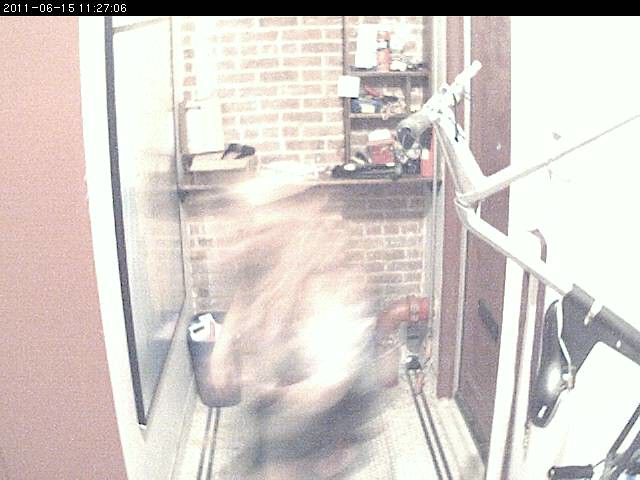In this image, we observe a narrow alcove, approximately three feet wide, featuring a backdrop of a brick wall. The floor appears to be covered with carpet or tile, although the exact material is unclear. On the right side of the alcove, a metal contraption is visible near the viewer. Affixed to the brick wall is a shelf cluttered with various items stored in small cubbies, along with some additional objects, including a box, stacked in a somewhat messy arrangement. A trash can is positioned against the left side of the brick wall. Near the bottom right of the wall, a red pipe emerges and descends into the floor. On the left wall, there is a framed picture or possibly a map. In the blurry foreground, a figure can be seen wearing what seems to be a white shirt, a vest, and either a helmet or a baseball cap, although the details are indiscernible due to the blurriness of the image.